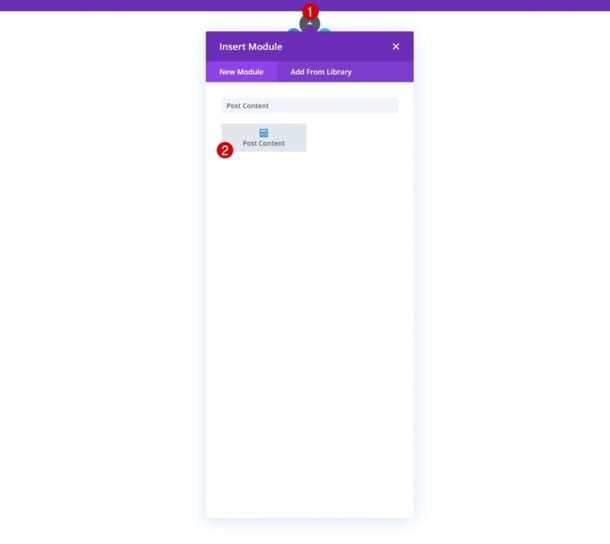Here is a cleaned-up and detailed caption for the image:

---

This screenshot captures a desktop interface of a graphical application, focused on module management. The main area showcases an infographic with a two-step process for inserting a module. 

1. **Insert Module**: On the left side, there is a button labeled "Insert Module," which is highlighted with a royal purple color. Adjacent to this button is a red circle containing the white numeral "1".
2. **Post Content**: To the right, there's another directive labeled "Post Content," rendered in dark gray text. It is marked by a red circle with the white numeral "2".

Additionally, within the "Insert Module" section, a partially obscured blue plus sign button is visible, suggesting the option to add new content or elements, though it is overlapped by the "Insert Module" window and the numerical indicator. The entire background of the interface remains a blank white canvas, indicating that content needs to be added through the specified steps.

At the top of the screenshot is a royal purple bar, matching the color of the "Insert Module" button, providing a cohesive visual theme to the interface. 

Overall, the interface appears empty and awaits user interaction to populate modules and post content through the specified sequential process.

---